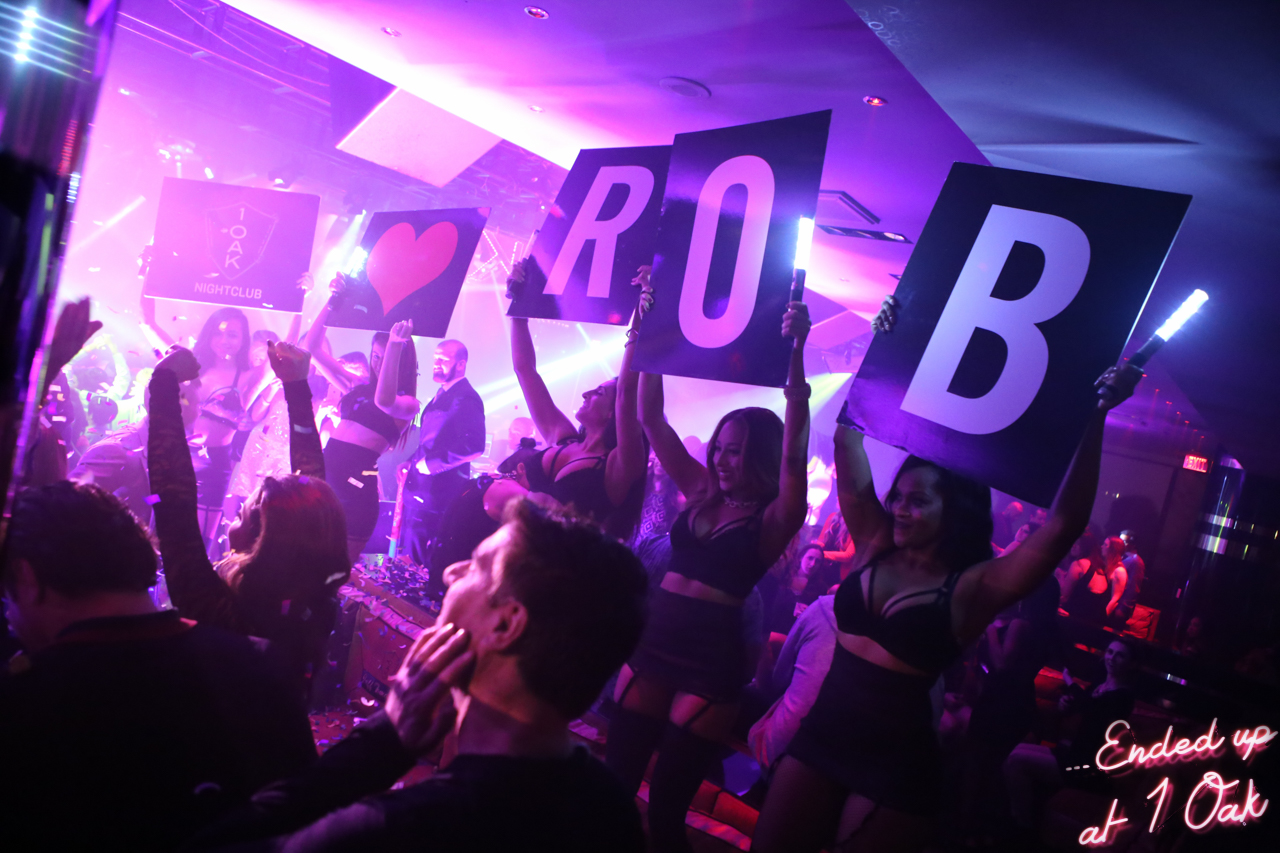In this vibrant, smoky pink-lit nightclub, a dynamic group of five women stands out amidst a lively crowd. Dressed uniformly in short black skirts and black crop tops, they hold up a series of black signs adorned with white and red lettering. From left to right, the signs spell out a heartfelt message: the first sign features a shield emblem with "One Oak Nightclub," the second sign displays a large red heart, and the following three signs spell out "ROB" in capital letters, forming the message "One Oak Loves Rob." Each woman holds a glow stick or flashlight rod, amplifying the celebratory atmosphere. Confetti floats through the air, suggesting a festive occasion. The pink stage lights and sporadic lasers enhance the club's energetic ambiance, while the crowded scene with cheering patrons and a few raised hands reflects the party’s enthusiasm. The final touch of the digital script text at the bottom right of the image reads, "...ended up at One Oak."